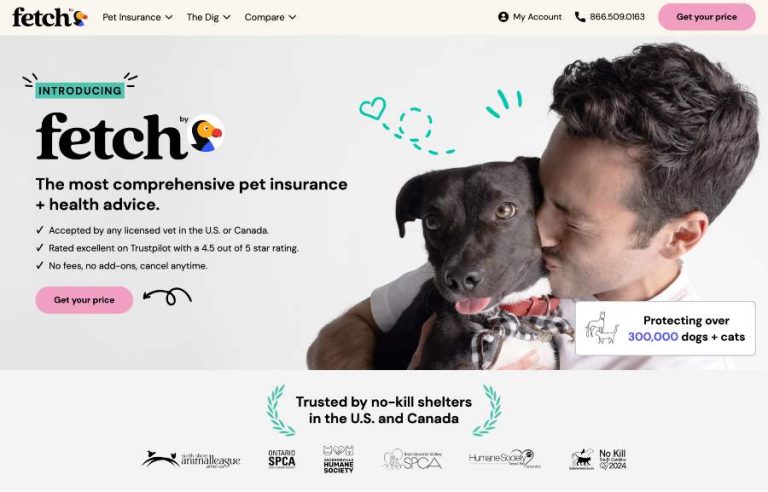The image appears to be a screenshot from a website. At the top, the header labeled "Fetch" is prominently displayed alongside a logo of a bird featuring a black head, a yellow face, and an orange beak. To the right of this header are three dropdown menus labeled "Pet Insurance," "The Dig," and "Compare." Further to the right, you can see options for "My Account," a contact phone number, and a pink button labeled "Get Your Price."

The main portion of the screen is divided into two sections with a gray background. On the left side, there is text enclosed within a green-bordered box that starts with the word "Introducing." Below this, the "Fetch" logo with the bird is displayed, followed by the tagline "The most comprehensive pet insurance plus health advice." Three check-marked statements are listed underneath:
1. "Accepted by any licensed vet in the U.S. or Canada"
2. "Rated excellent on Trustpilot with a 4.5 out of 5 star rating"
3. "No fees, no add-ons, cancel any time"

Below these statements, there is another pink "Get Your Price" button.

On the right side of the screen, there is an image of a man holding a brown dog. The man appears to be giving the dog a kiss on the head. He has short brown hair, and the dog, which has brown fur and brown eyes, is facing forward with its tongue sticking out and wearing a red collar.